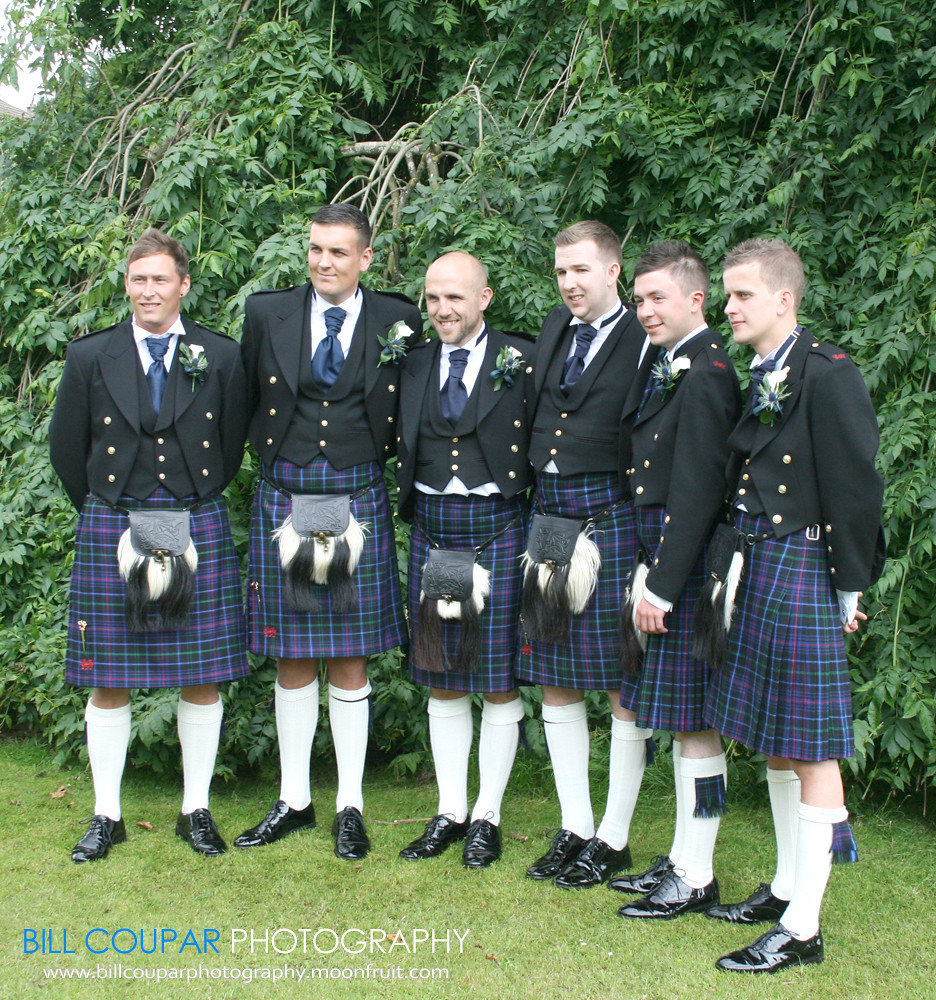The image captures six men arranged in a slight half-circle, looking towards the left side of the frame. They are dressed in formal black jackets with shiny metallic buttons, black waistcoats, white shirts, and blue ties, each accented with a flower pin on their lapels. They are all wearing traditional Scottish kilts in a blue, green, and red tartan pattern, complemented by white knee-length socks and polished black dress shoes. In front of each kilt is a sporran, a grayish-black pouch adorned with white and black hair. The men stand on a patch of green grass, with lush overgrown trees and vegetation serving as a natural backdrop. The bottom left corner of the image displays the text "Bill Kupar Photography" and the website "www.billkuparphotography.moonfruit.com," suggesting the photo's professional origin. The coordinated attire and the formal nature of the setting imply that they are likely groomsmen at a wedding.